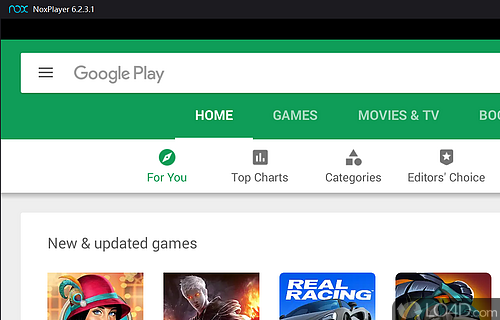This screenshot captures the interface of the Google Play store. At the top, we see the "Google Play" logo accompanied by a search bar. Directly beneath are navigation tabs labeled "Home," "Games," "Movies & TV," and "Books." Further down, the section headers read "For You," "Top Charts," "Categories," and "Editor's Choice." The main area showcases the "New & Updated Games" section featuring partial images of several games. The first image displays a woman wearing a hat, partially obscured to show only a segment of her face. The following image is an artistic drawing likely depicting a man. The next game, titled "Real Racing," reveals a portion of a Formula race car. The subsequent image is more ambiguous, featuring a mix of green, black, and other colors set against an orange background, with the text at the bottom stating "load.com." The header at the top of the screenshot indicates the user is operating within "Knox Player 6.2.3.1." The primary color scheme includes a green header bar, white background, and various colors from the game images.